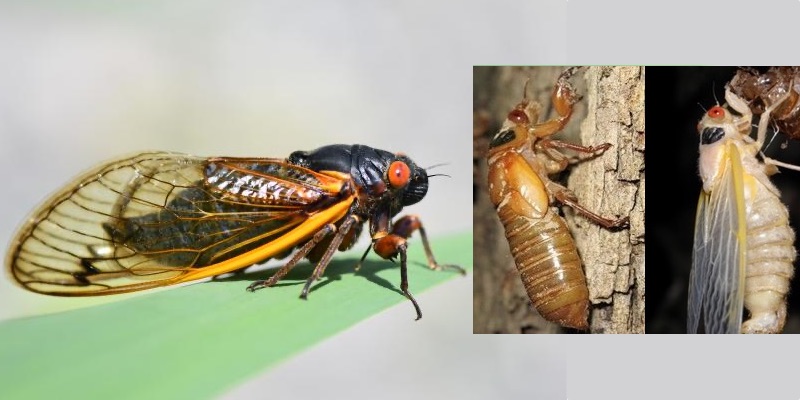The image is a detailed photorealistic depiction of cicadas, divided into three sections. The left half showcases a close-up of a mature cicada with a black body and striking deep red eyes. It is standing on a long green leaf, displaying its four visible legs and transparent orange-tinted wings, with intricate veins clearly visible, against a gray background. To the right, two smaller photographs illustrate different stages of the cicada's development. The middle photograph features a cicada with a lighter brown, almost caramel-colored body, clinging to the white bark of a tree, and it appears to lack wings, indicating an earlier stage in its lifecycle. The rightmost photograph displays a cicada with a cream-colored body, beginning to emerge from its shell, attached to a small pine cone. This latter stage exhibits delicate, white wings bordered in yellow. Both of these cicadas also have red eyes, with the rightmost image having more vibrant colors, possibly suggesting it is depicted at nighttime.